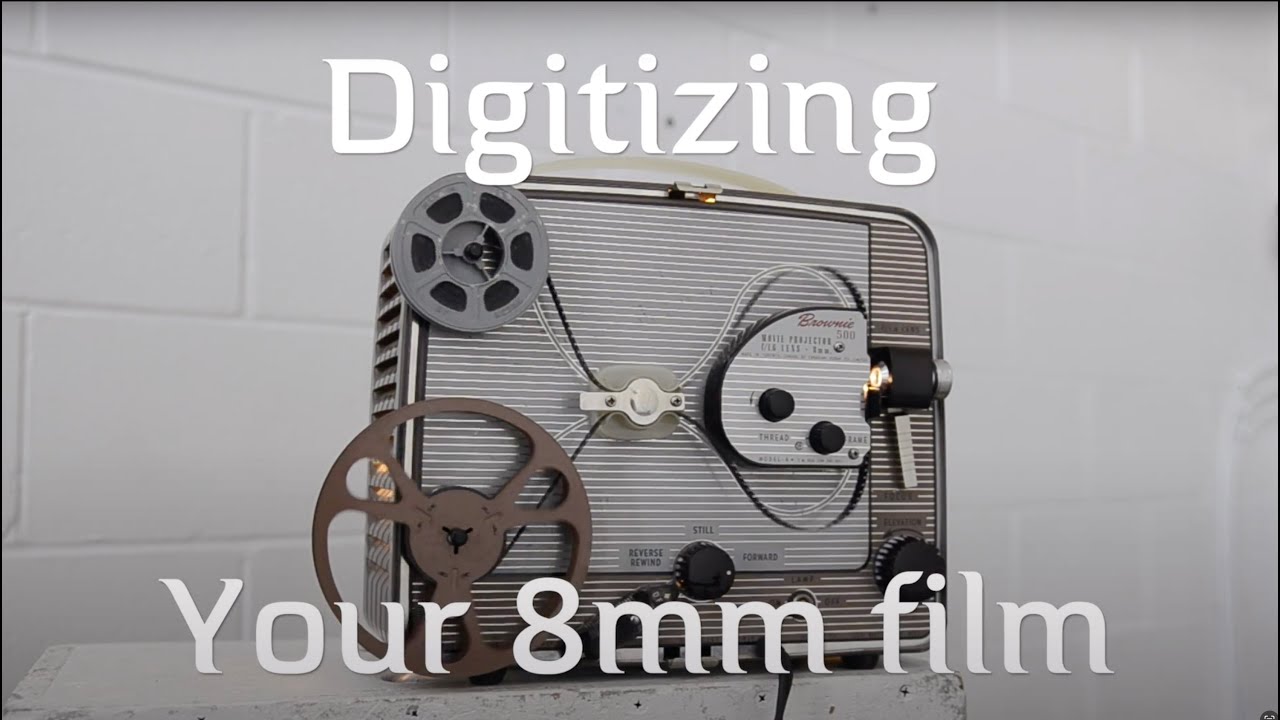The image captures a close-up of a vintage movie projector, prominently showcasing its light tan and olive green metal body. The projector is oriented at an angle, revealing the left side and front, but not the back. Central to the scene are two reels: a large cream-colored reel at the bottom and a smaller black reel above it, both with film winding between them. The film threads through a white plastic attachment and arcs around a half-circle area, feeding towards a prominent circular lens on the right side of the projector where the light emits. Behind the lens are a couple of control knobs.

A set of hands is interactively threading the film; one hand is positioned under the light area, delicately touching the film, while the other hand is atop the projector, pinching the film with the thumb and pointer finger, suggesting an attempt to properly feed the film through the machine.

The projector rests on an aged, worn wooden box, its paint chipping away, indicative of its long-term use. The background is blurred but reveals a white floor leading to a dark wall, a white wall, and a possible entryway. This intricate scene highlights the meticulous process involved in setting up the film on such a classic device, reflecting the charm and complexity of vintage cinematography equipment.